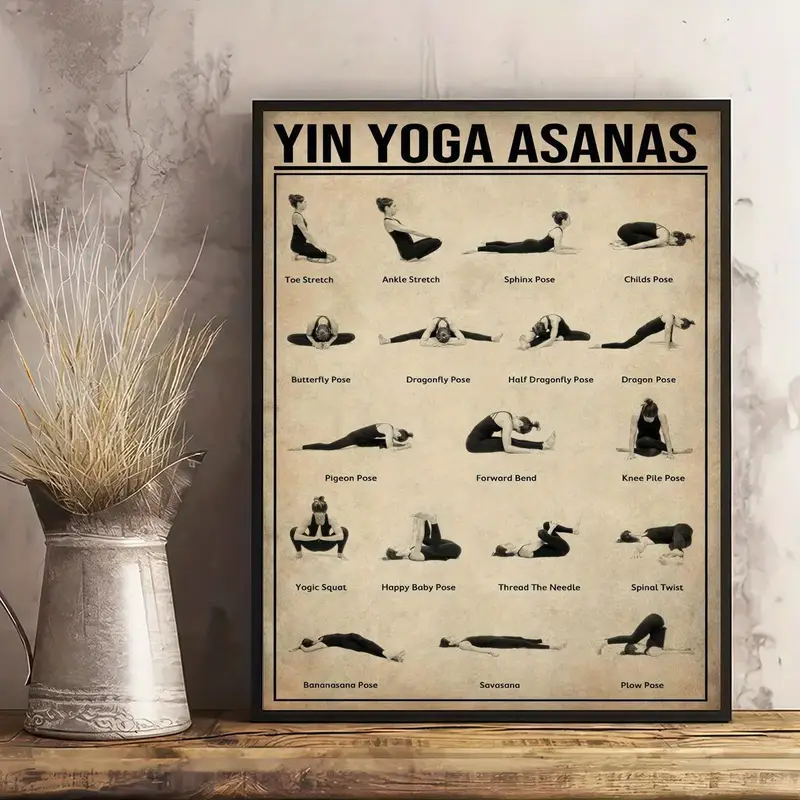The photo shows a vintage-inspired decorative scene featuring a horizontal-grained wooden surface, likely a shelf or table, against a white wall with slight dark gray discoloration. Leaning against the wall is a poster displayed in a black frame. The poster, titled "Yin Yoga Asanas" in bold black letters at the top, displays multiple yoga poses including toe stretch, ankle stretch, sphinx pose, child's pose, butterfly pose, dragonfly pose, half dragonfly pose, dragon pose, pigeon pose, forward bend, and kneel pile pose, among others. Each pose is individually outlined within a large black rectangle. To the left of the poster sits an old-fashioned tin pitcher, possibly repurposed from an ash can or metal watering pot, filled with decorative dried brown grass or hay sticks. The overall scene is complemented by light mauve wallpaper in the background, enhancing the serene and vintage ambiance.